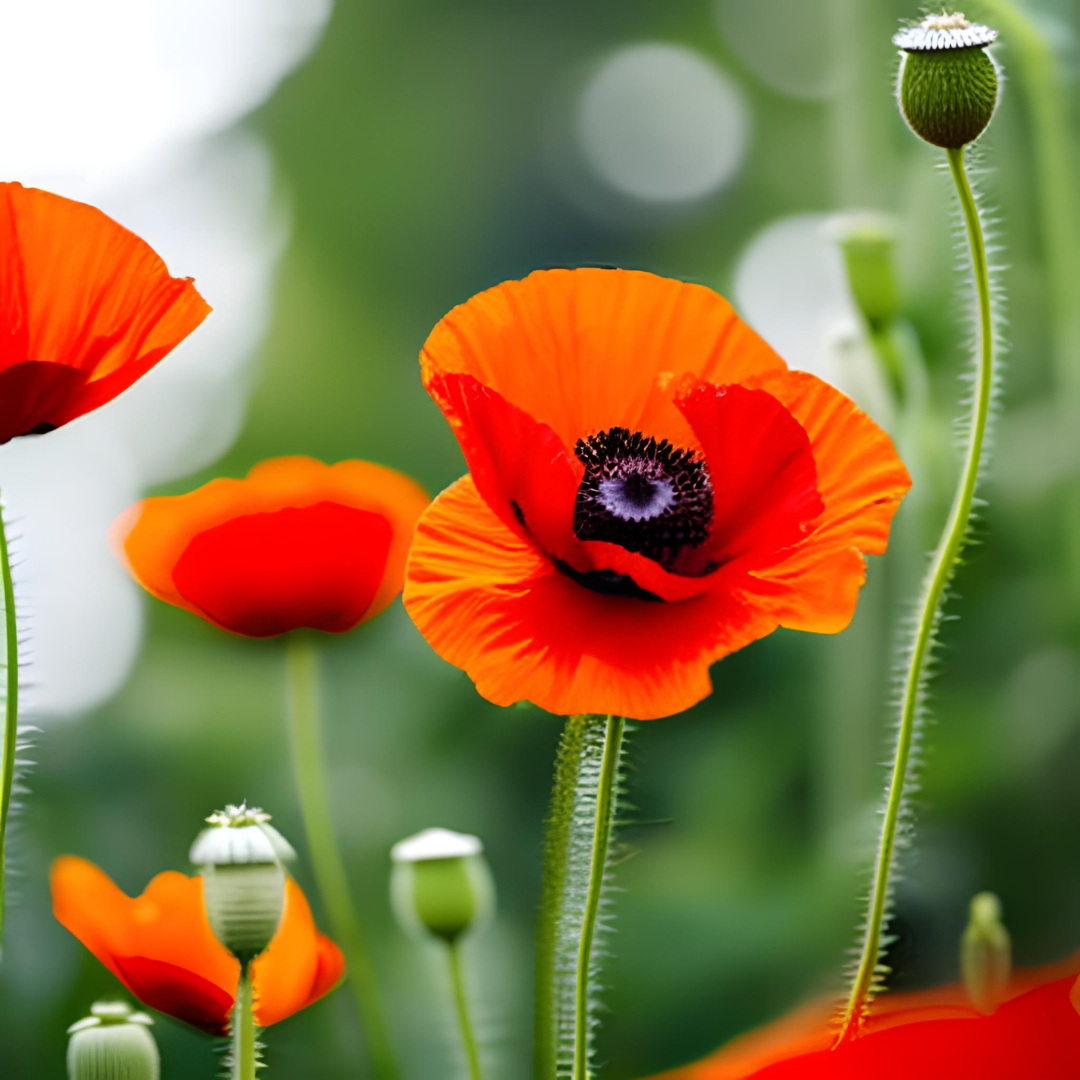This photograph, taken outside, features a close-up of an orange poppy flower just slightly right of center. The flower stands prominently with layered orange petals—one layer on top and another beneath—surrounding a center composed of small black buds, a light blue inner circle, and an innermost black core. Its green stem, adorned with white hairs, curves slightly before reaching up to support the bloom. To the left, blurred background elements reveal more orange poppies and unopened green buds. Notably, the very left edge of the image shows another orange poppy in clearer focus. On the right, a tall green stem with a yet-to-bloom pod extends above the central flower. The background hints at greenery, potentially trees and bushes, with some white specks that might be flowers. The bottom right corner of the photograph also captures a slightly out-of-focus petal, matching the orange hue of the central poppy.